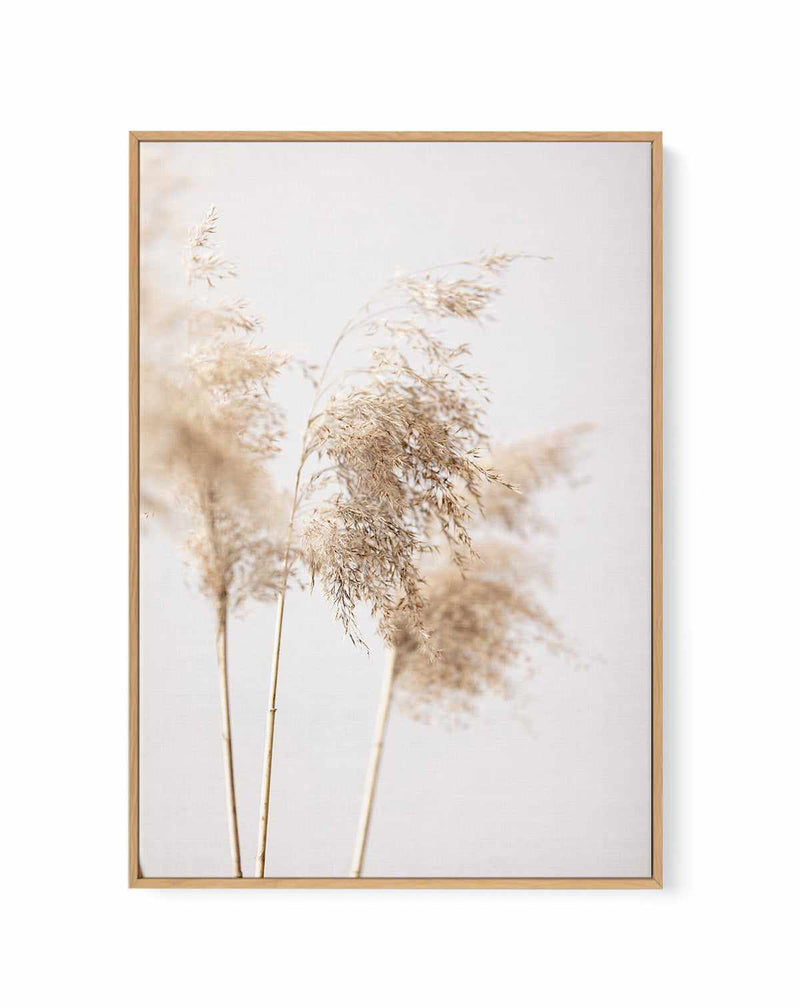This is a highly detailed, vertical rectangular photograph showcased within a large, natural-colored wooden frame. The photograph itself is set against a very light grayish, cream-colored background. At the center of this composition, there are three dried stems, each topped with a wheat-like seed head, which stand tall but tilt slightly to the right. The seed heads, akin to the intricate puffs of pampas grass, exhibit a soft, tannish-golden hue. The two seed heads on the left and right are out of focus, creating a blurred effect, while the central seed head remains sharply in focus, revealing its delicate, tiny details. The artwork captures the fragile essence of these ornamental grasses, with the sharpness of the central seed head highlighting its texture, which would likely crunch if squeezed, contrasting with the softer, dream-like appearance of the flanking stalks.